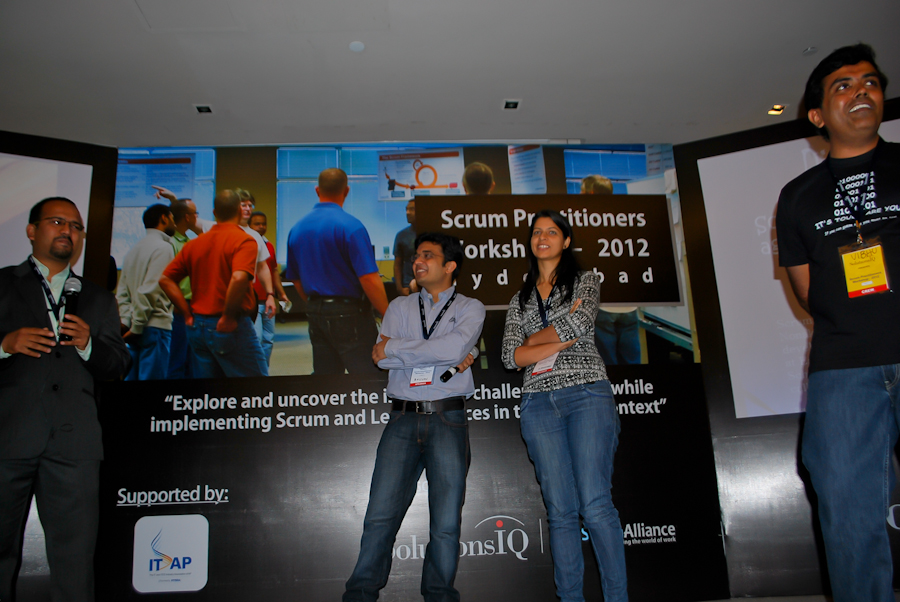The photograph captures a lively scene where four people are gathered on a stage. The backboard behind them is partially obscured but reads "Scrum Practitioners, Yorkshire 2012," supported by ITAP and Solutions IQ. On the far left, an older man in his 30s is wearing a black suit, eyeglasses, and a black name tag lanyard as he speaks into a microphone. To his right, an Indian woman with long black hair, wearing a black and white blouse and blue jeans, stands smiling with a black name tag around her neck. Next to her stands another Indian man, dressed in a blue button-down shirt and jeans, holding a microphone. Further to the right, almost out of the picture, a man in a black t-shirt with white writing, blue jeans, and a black lanyard smiles brightly. Above them, a white ceiling frames the scene. The mood is celebratory, suggesting that the presentation involved good news or achievements, as evidenced by the shared smiles and engaging interaction.